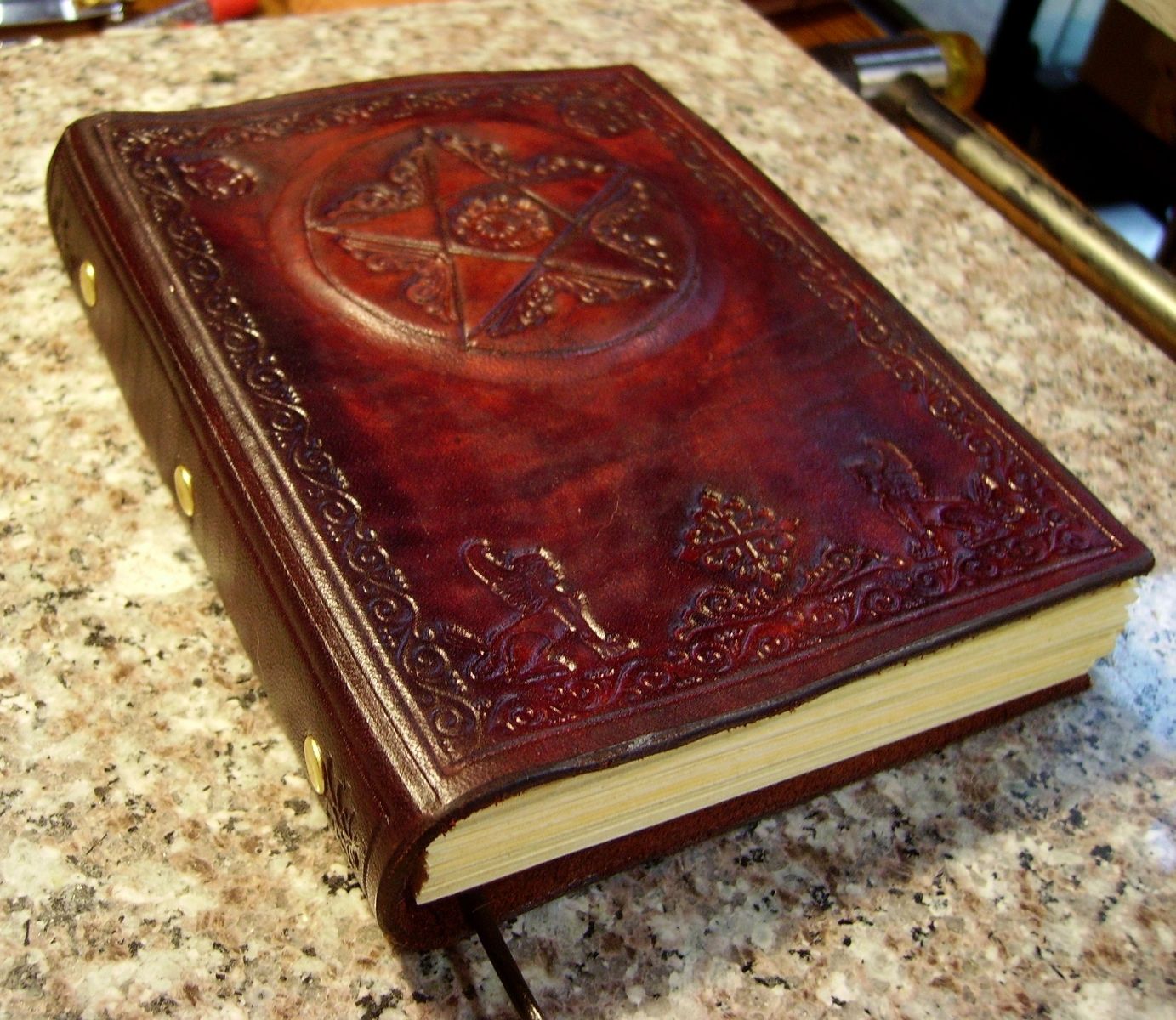This photograph captures an ancient, intricately-designed book placed centrally on a marbled surface, which likely resembles a brown, white, and black granite countertop. The book is imposing and thick, suggesting it contains hundreds of pages. Its cover, crafted from a reddish-burgundy leather, is adorned with detailed etchings and symbols. The centerpiece of the cover features a prominent, elaborate pentagram enclosed within a circle, evoking a sense of dark, arcane mysticism. Surrounding the pentagram, floral patterns adorn the four corners, while the bottom boasts scrollwork and depictions of creatures guarding a cross-like structure. The book's spine is reinforced with three brass tacks, indicating its sturdy construction. Additionally, a black bookmark emerges from its pages. To the right, partly off the marbled surface, an object, possibly a metal hammer, adds to the mysterious ambiance of the scene.